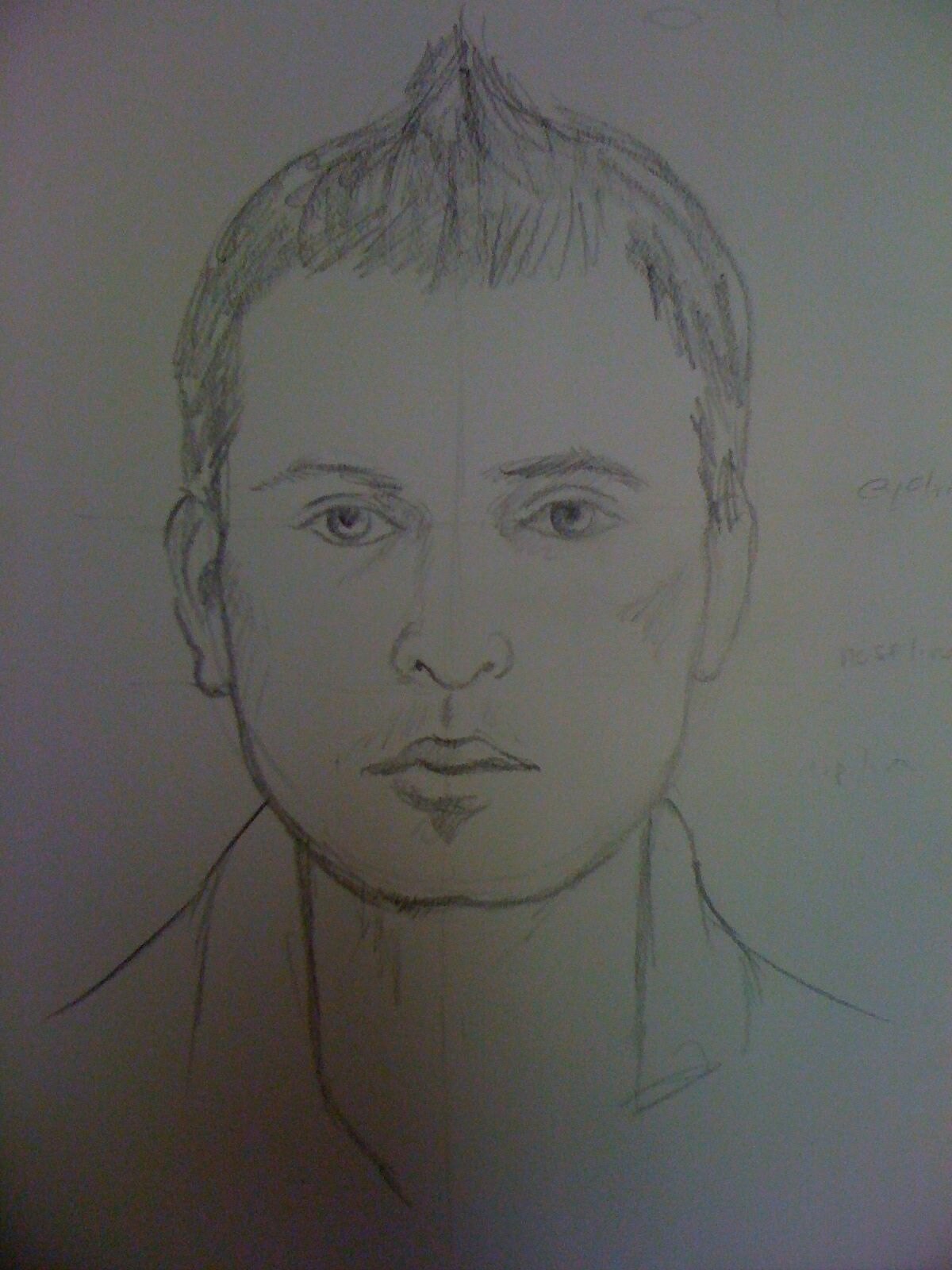The image is a pencil drawing on a blank white sheet of paper, featuring a detailed portrait of a man. Taken in a dimly lit space, the sketch is slightly unclear but reveals a range of facial features: expressive eyebrows, eyes, a button nose, medium-sized lips, and a hint of stubble above and below the lips. The man has a short mohawk hairstyle, with the sketch extending down to just above his shoulders, where he appears to be wearing an open-collared shirt. Guideline marks are visible on the face, aiding in symmetry, and notes indicate positions for the eyes, nose, and mouth along a grid. The drawing is entirely monochrome, using only pencil, and emphasizes the man's direct gaze towards the viewer.